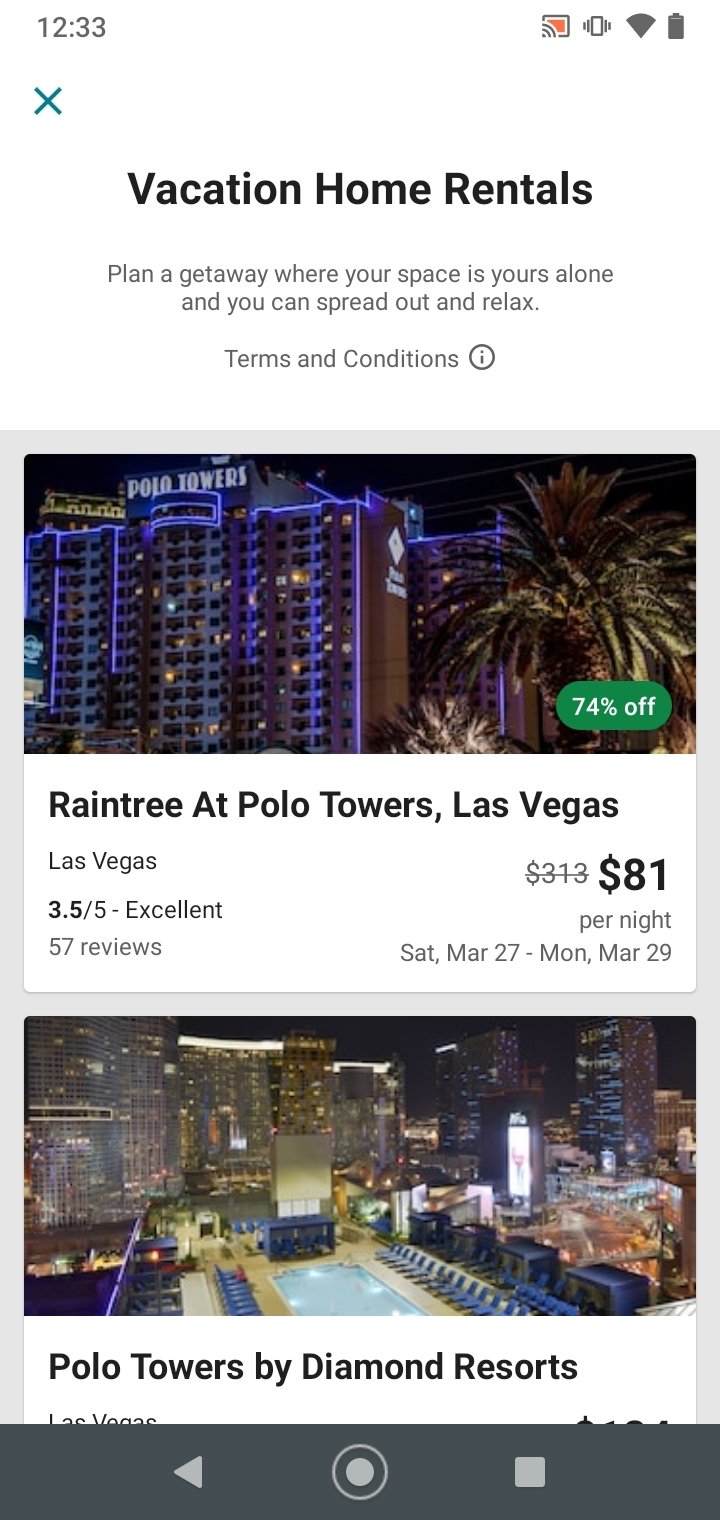The image appears to be a promotional screenshot taken from a smartphone, most likely from either an iPhone or an Android device. It showcases a detailed advertisement for vacation home rentals. 

**Top Section:**
- **Time and Icons:** 
  - The top section, upper left, displays the time "12:33" in black.
  - The upper right corner features several icons: an orange and gray Wi-Fi icon, another gray and white icon which resembles a network indicator, and a full battery logo.

**Main Ad Content:**
- **Header and Subheader:**
  - Immediately below the time, there's a blue 'X' symbol.
  - Centered below that in black lettering, it states "Vacation Home Rentals."
  - Further below, in smaller black letters, it reads: "Plan to get away, where your space is yours alone, and you can spread out and relax."
  - Following that, the phrase "Terms and conditions" is noted, next to a gray circular icon with a gray letter 'i' inside.

- **Property Details:**
  - The top part is outlined in gray on the top and sides, containing images of Las Vegas properties.
  - **Top Rectangular Image:**
    - A nighttime photograph of a tall building labeled "Polo Towers" in white letters.
    - The building features blue lighting along its sides and has a large date palm tree to the right.
    - In the lower right of this image, there's a green oval with "74% off" in white text.
  - Information below the image includes:
    - A white bar with "Rain Tree at Polo Towers, Las Vegas" in black letters.
    - "Las Vegas" is written to the right of that.
    - The rating "3.5/5, Excellent" followed by "57 reviews" in gray.
    - A crossed-out price of "$313" replaced by "$81 per night" in bold black text, with "per night" in gray below.
    - The dates "Sat, Mar 27 - Mon, Mar 29" separated by a gray area.

- **Lower Rectangular Image:**
  - Another nighttime image displaying a large resort all lit up, with what appears to be a pool in the lower center.
  - "Polo Towers by Diamond Resorts" is prominently displayed in black letters on a white background.
  - "Las Vegas" is partially visible to the lower left but gets cut off at the bottom.

**Bottom Section:**
- **Navigation Bar:**
  - The very bottom features a long gray bar with controls for media navigation:
    - A gray circular play button that includes a darker gray circle inside, containing a lighter gray circle in the middle, resembling a stop button.
    - To the right of this play button, there's a gray square.